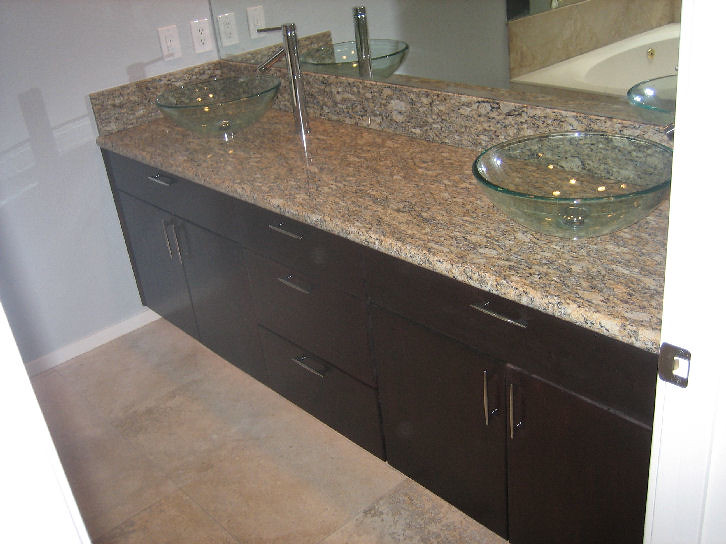This image showcases a luxurious and modern bathroom countertop that appears to be part of a newly constructed high-end bath sink unit. The countertop boasts a sleek, nearly black marble stone surface that exudes sophistication. Mounted on the counter are two elegant, clear glass vessel sinks, each shaped like a bowl and anchored at their small bases, revealing the drains at their centers.

The faucet above each sink features a contemporary design, characterized by high arching spouts with single-lever controls and a down-slanted spout, a popular choice for modern fixtures. A matching faucet can be seen peeking from the right side of the image, hinting at the symmetrical design of the bathroom.

The mirror on the wall reflects a high-end bathtub equipped with side-mounted jets, adding to the luxurious feel. The side of the tub and the splash area share the same marble stone look as the countertop, though with a different pattern, creating a cohesive aesthetic. The countertop drawers are adorned with attractive, narrow metallic handles that have a stylish pewter finish.

The flooring in the bathroom features large tiles with very thin grout lines, offering a seamless and expansive appearance. The room is completed with light-colored baseboards and walls painted in a soft gray, punctuated by several modern fixtures mounted beside the bath unit. This image captures the essence of contemporary elegance and sophisticated interior design.